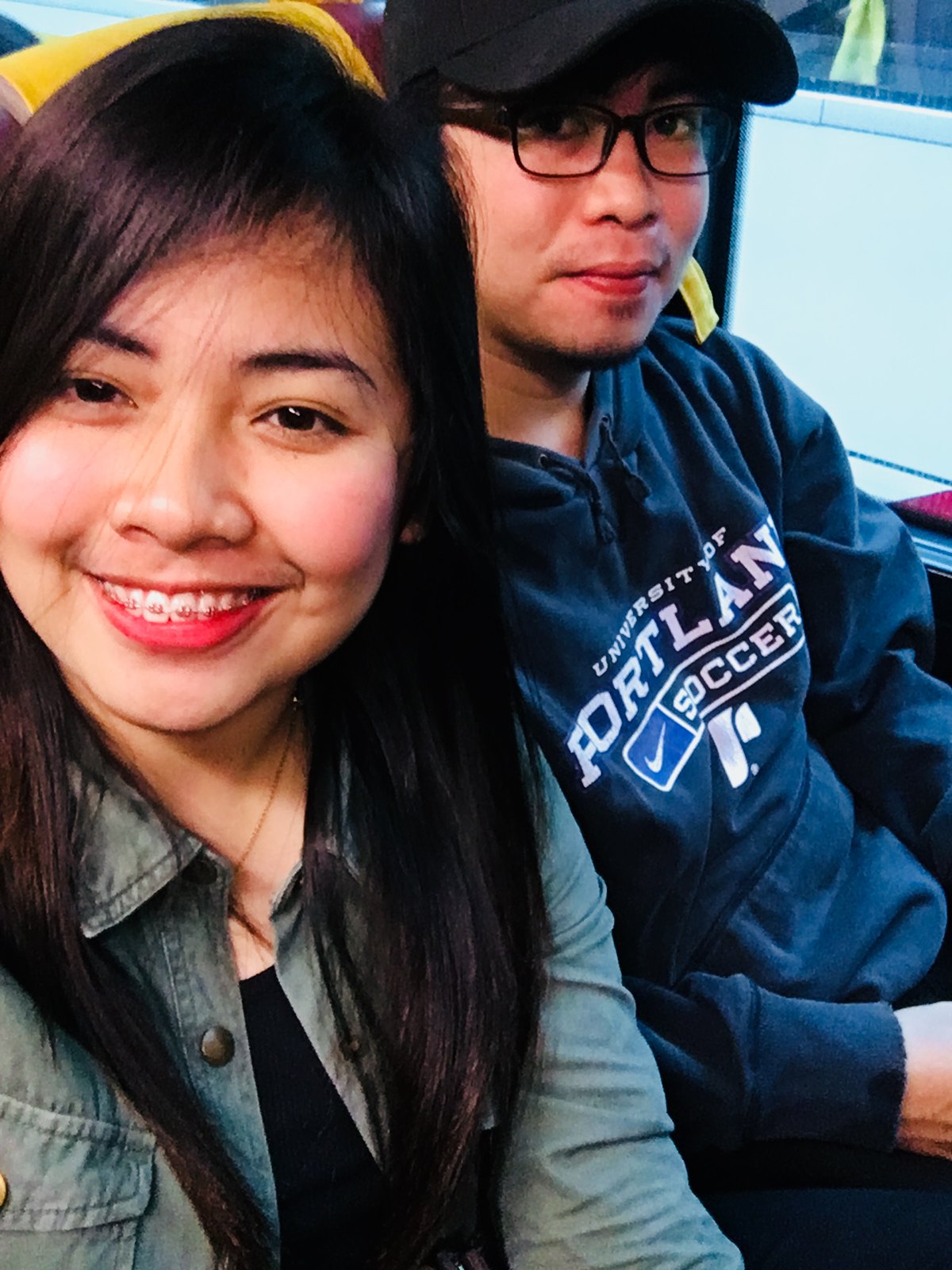This is a vibrant color photograph capturing a selfie of a young Asian woman and an Asian man, likely on public transportation such as a bus or train, evident from the yellow seats behind them and a large window by the man's side. The woman, positioned on the left, is beaming with a bright smile, showcasing her braces. She has long, straight black hair and is dressed in a black t-shirt layered with a denim jacket. Next to her, the man exudes a more reserved demeanor, gazing at the camera without a smile. He sports a black tracksuit with sweatpants, a black baseball cap, and black rectangular glasses. His sweatshirt features the words 'University of Portland Soccer' along with a Nike emblem, suggesting he might be associated with the university. The man also has a beard and mustache, adding a slight maturity to his appearance.